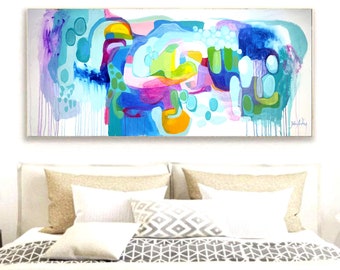This detailed description captures the essence of the photograph, emphasizing shared and repeated elements:

The photograph depicts a cozy bedroom with a bed pushed up against a pristine white wall. The bed features a white headboard and is adorned with an assortment of pillows, including brown, white, and gray chevron pattern pillows. Notably, there is a pillow that is slightly off-center to the left, adding a touch of imperfection to the arrangement. The gray and white patterned blankets are neatly pulled up to the row of pillows. Above the bed, perfectly aligned with the headboard, hangs an abstract painting on a white canvas. This vibrant artwork showcases a medley of bright colors such as blue, pink, green, orange, and purple. The colors form rounded shapes reminiscent of bubbles, with some elements appearing to drip down towards the bottom of the canvas, blending together to create a striking abstract piece.